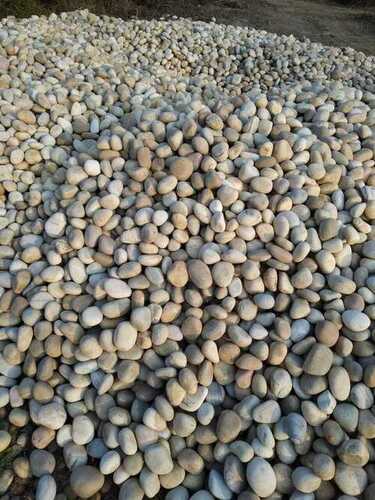A large pile of stones of varying sizes, resembling small eggs, is depicted in this outdoor image. The stones display a range of colors, including beige, dark gray, light gray, and brown. The majority of the stones are clustered densely in the center of the image, while they begin to thin out towards the edges. In the background, the stones give way to bare ground, suggesting the end of the pile. The overall scene highlights the assortment and natural arrangement of these stones in an open, likely outdoor environment.